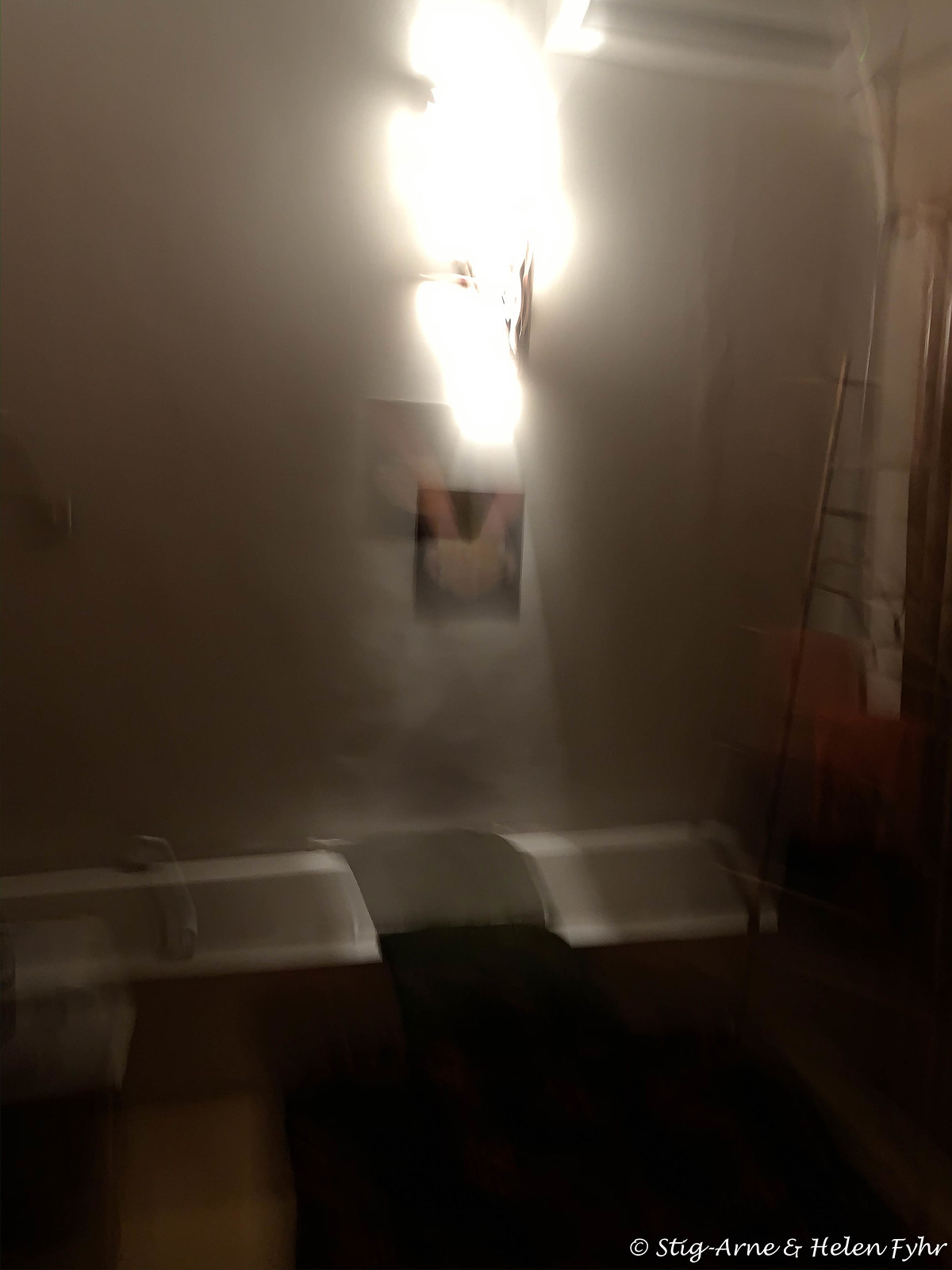The image depicts a partially renovated bathroom. In the foreground, there's a sink, possibly in the midst of reinstallation, with a reflection that adds to the visual complexity. A ladder is positioned nearby, suggesting ongoing renovation work. The scene is brightly illuminated by a strikingly luminous light source on the wall, which creates an ethereal effect, resembling a person suspended in mid-air. Further in the background, another bathroom fixture, potentially either a second sink or a tub, is visible. The floor appears to be covered with a tan-colored throw rug, adding a touch of warmth to the scene amidst the renovation chaos.